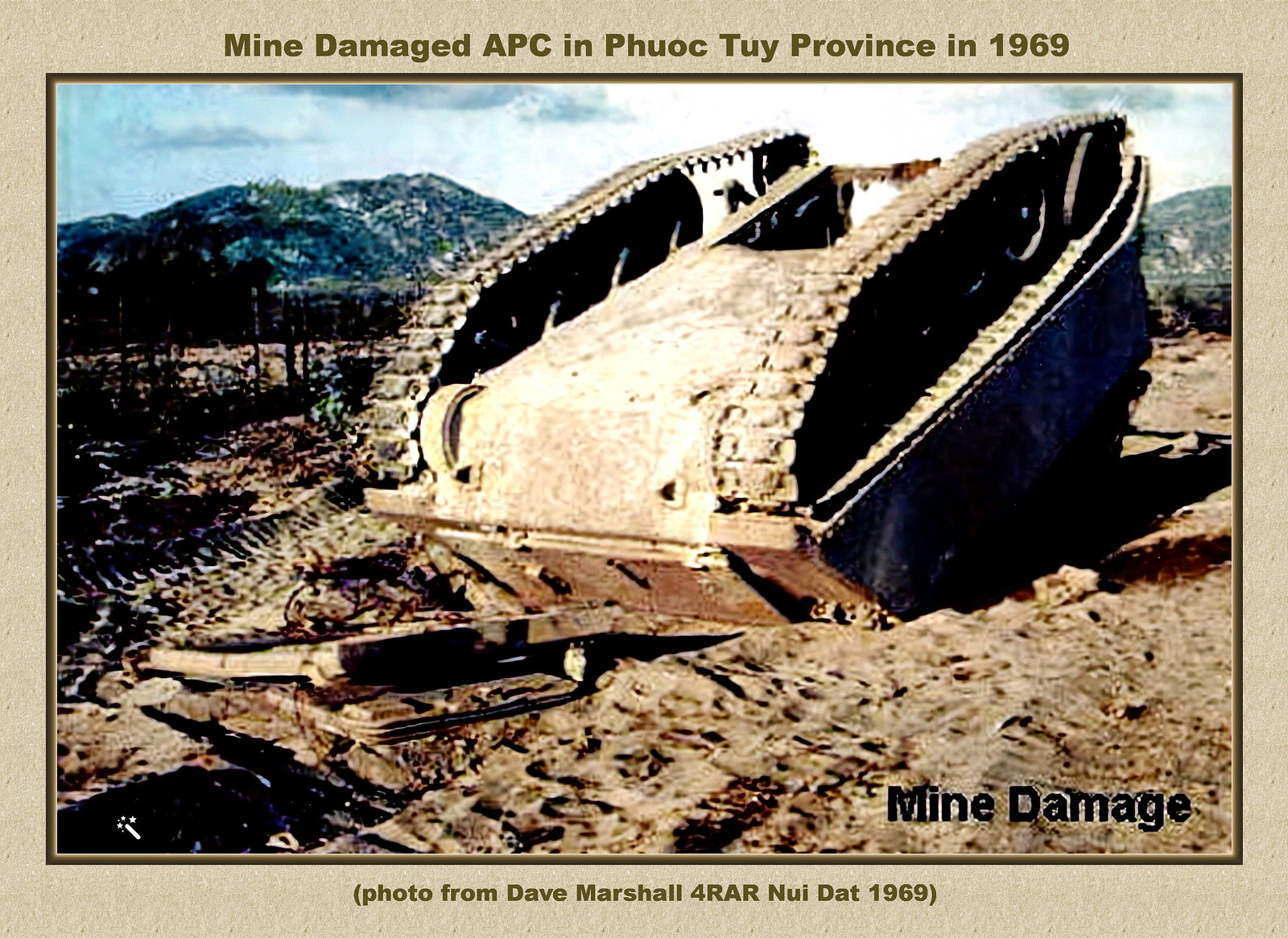The image depicts the aftermath of a mine-damaged APC (Armored Personnel Carrier) in Phuoc Toi province, Vietnam, taken in 1969. It has a light brown, granite-like background. At the top, the text reads: "Mine damaged APC in Phuoc Toi province in 1969," while the bottom states: "Photo from Dave Marshall for RAR Nui Dat 1969." The APC is shown upside down, exposing its tracks and underside, indicating it was overturned by an explosion. The scene is set on a dirt and sand terrain with mountains in the backdrop, under a cloudy sky. The photograph has a beige-tan tint, adding to the historical and grainy quality of the image. No people or animals are visible, emphasizing the desolation at the site of the explosion.